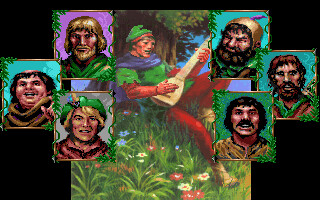The image appears to be a screenshot from a vintage computer video game. The central focus is on an intricately detailed main image featuring a male character situated in a lush, forested environment. He is seated on the ground amidst a vibrant array of plants and flowers, leaning against a towering tree. His attire is distinctly colorful: a green hat, a green shirt accented with red sleeves, red tights, brown boots, and matching red gloves. He is absorbed in playing a stringed instrument resembling a guitar or fiddle.

Flanking this main image are six smaller, overlapping portraits arranged in two vertical columns—three on each side. Each portrait showcases a different male character, evoking a sense of historical or fantasy settings. The left-hand column consists of three neatly arranged individual photos, while the right-hand column mirrors this arrangement with three more characters, each photo slightly overlapping the next. Together, these elements create a rich tapestry that suggests a scene from a past era, blending elements of pastoral serenity with detailed character design.